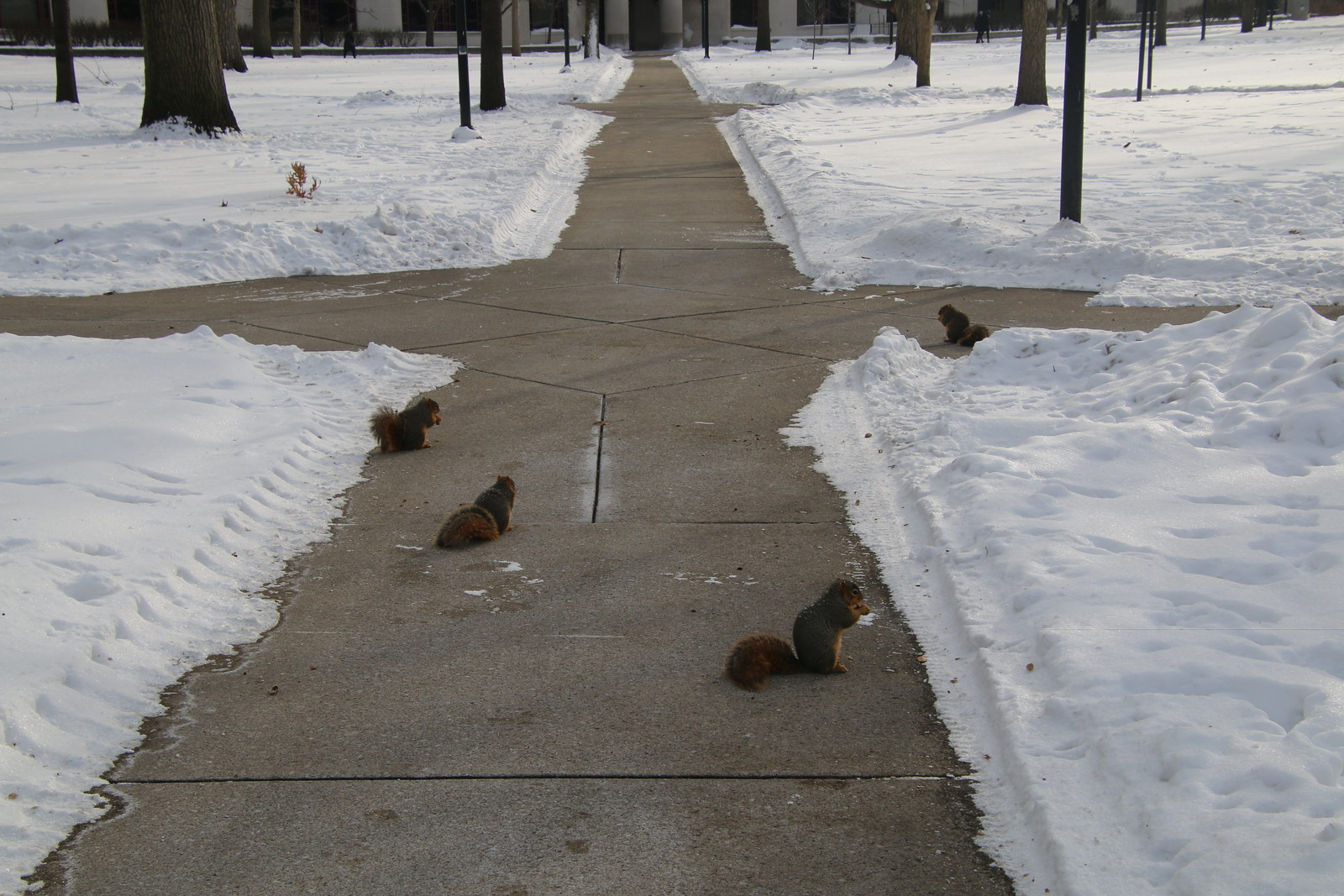The photograph captures a detailed winter scene featuring a heavily snowed area with a T-shaped intersection of two cleared sidewalks. The dark concrete of the sidewalks sharply contrasts with the deep white snow piled on either side. In the foreground, four brown squirrels occupy the cleared walkway, all sitting upright and appearing to eat something. One notable squirrel is perched on its back legs, holding a piece of snow in its paws as if puzzled by it. Another squirrel, with its tail fluffed up for warmth, is positioned on the left side of the sidewalk, gazing up the path. The remaining two squirrels are dispersed along the horizontal stretch of the intersection, each engaged in nibbling what they have found. The background reveals the base of a commercial building and dark tree trunks of varying sizes, from thin to a notably hefty trunk on the left. This color photograph, wider than it is tall, is devoid of people, writing, or vehicles, focusing solely on the serene winter landscape and the curious actions of the squirrels.